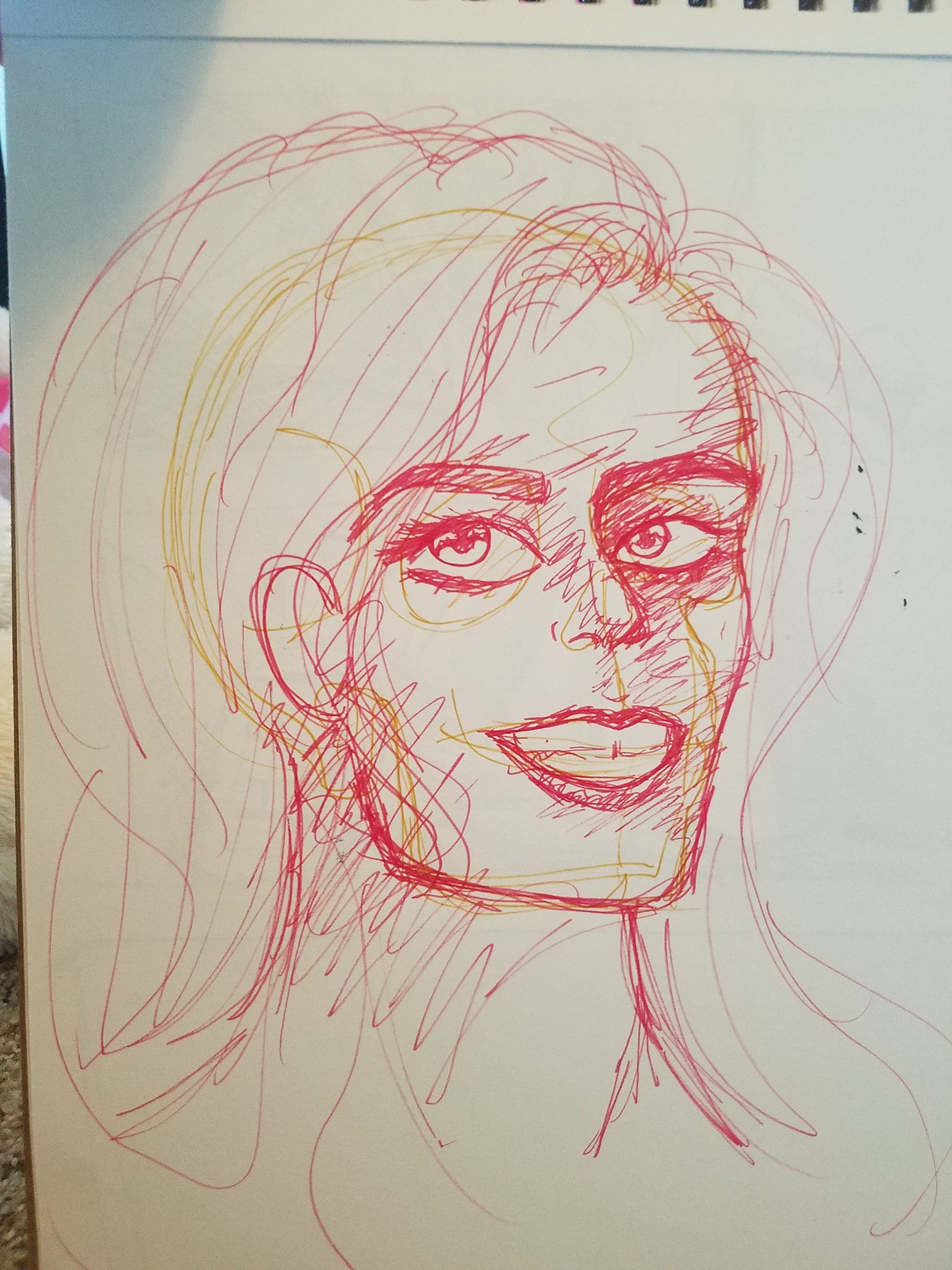This image portrays an early-stage sketch, meticulously outlined with what seems to be a felt marker or colored pencils. Dominantly featuring vivid red hues, the sketch also incorporates generous touches of yellow. The subject appears to be a woman, captured smiling warmly and gazing directly at the viewer. Her hair, medium-length and casually draped over her shoulders, suggests an effortless elegance. The background is an off-white canvas, with a visible crease at the top, hinting at other sheets of paper being flipped behind it. The woman's facial features are delicately rendered, emphasizing her small, defined nose, expressive large eyes, and prominent, thick eyebrows, adding character and depth to the nascent artwork.